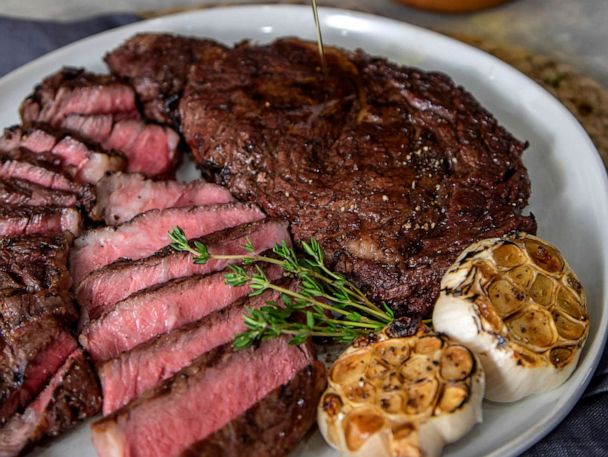A delectable steak dish is presented on a circular white plate, which sits atop a wooden table. Dominating the upper right portion of the plate is a large piece of steak, predominantly brown with a hint of black char marks. A toothpick protrudes from its center. Nestled below the steak in the bottom right are halved and baked onions, their white bases transitioning to a blend of brown and black on their roasted tops. Scattered small circles suggest intricate seasoning. Above these onions and slightly to the left, a singular green stem with tiny green leaf vegetables adds a touch of freshness, lying gracefully over the dish. On the left side of the plate, an array of steak slices, brown on the outside and revealing a pink, medium-rare center, spread out enticingly. This impressive assortment includes roughly 17 or 18 pieces, including several potential cuts like filet or Charlotte. The vibrant contrast of the pinkish-red meat against the plate enhances the visual appeal, making this steak dish both a visual and culinary delight.